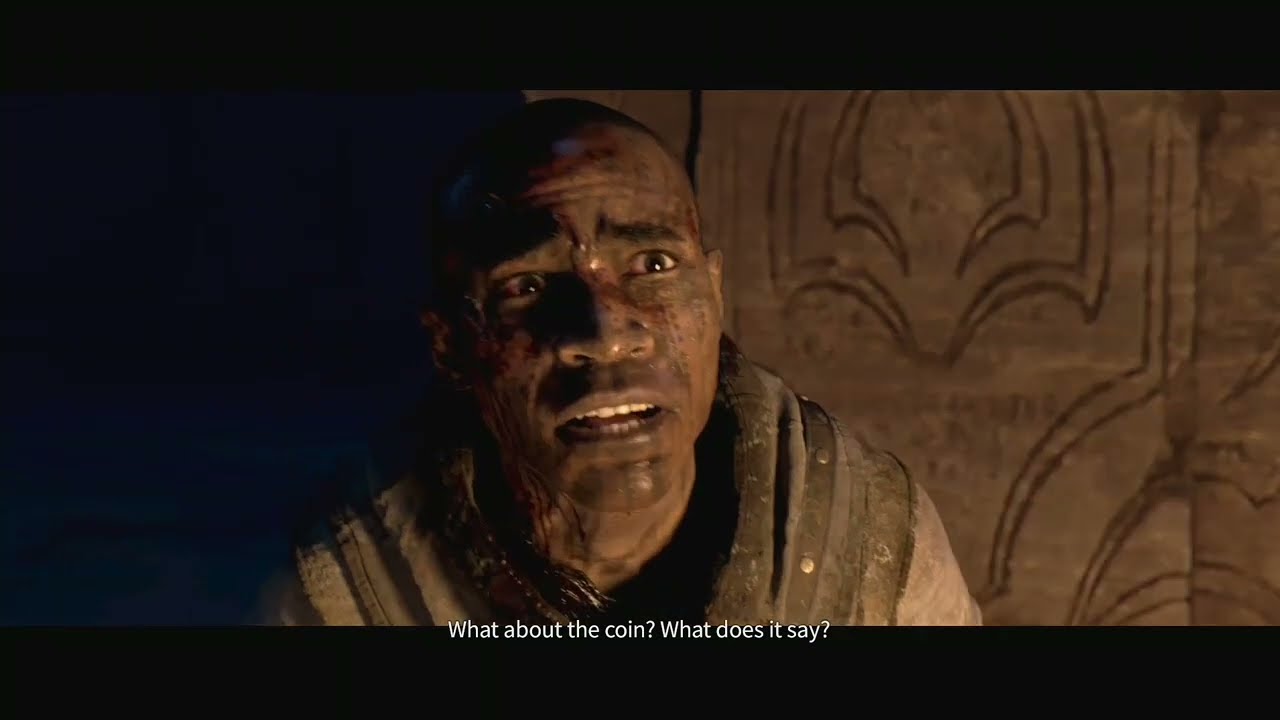The image is a digitally created scene depicting a distressed man sitting at the center. The man has dark, grimy skin contrasted by his white teeth, and dark short hair with a balding spot on top. Blood is seen trickling down the right side of his face, while light highlights the left side, revealing his fearful expression with an open mouth, exposed teeth, furrowed brow, and crinkled forehead. He wears a tattered, dirty robe in shades of gray, black, and white. Behind him, there is a dark gray stone wall etched with geometric brown patterns. To the left, there seems to be a night scene or dimly lit exterior visible through an opening. The bottom of the image is overlaid with the text, "What about the coin? What does it say?"